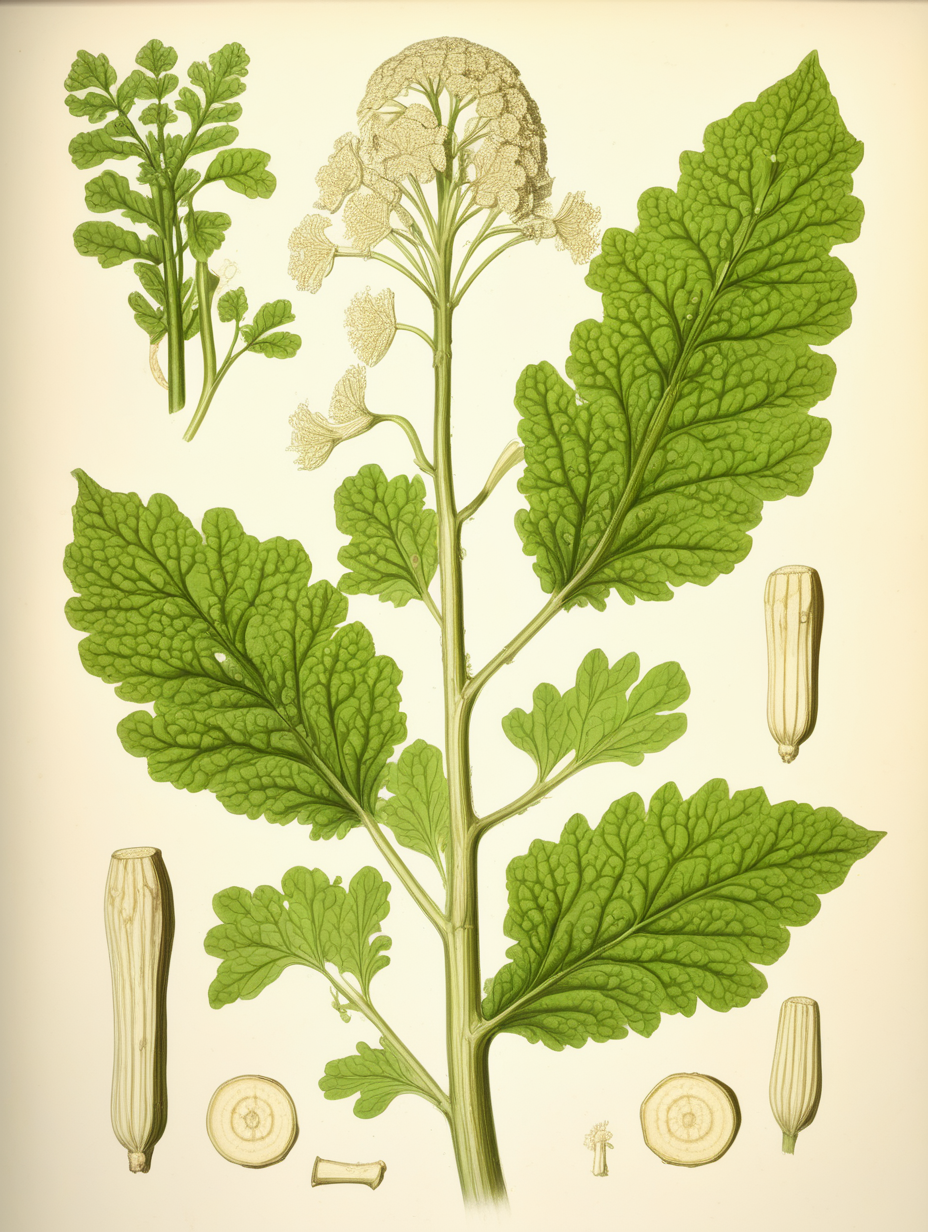This image appears to be a botanical illustration, possibly from a vintage textbook, and features a meticulously detailed drawing of a plant against a pale parchment-like background with darker edges. Central to the image is a long green stem that prominently branches out into multiple sections. At the top of this stem, delicate cream-colored flowers with many fine petals are depicted, resembling unopened tubular buds. The leaves, scattered along the length of the stem, are various sizes with noticeable bumps and scalloped edges. On the right, there's a sizable green leaf, mirrored on the left by another large leaf, while smaller leaves cluster towards the bottom and right side. Complementing this main composition, the top left corner showcases a sprig of green plants, detailed with mint-like foliage though not triangular in shape. The drawing eloquently captures both the botanical features, including presumed fruits alongside the leaves, and the vintage aesthetic of the background, contributing to a textured beige-green color palette.